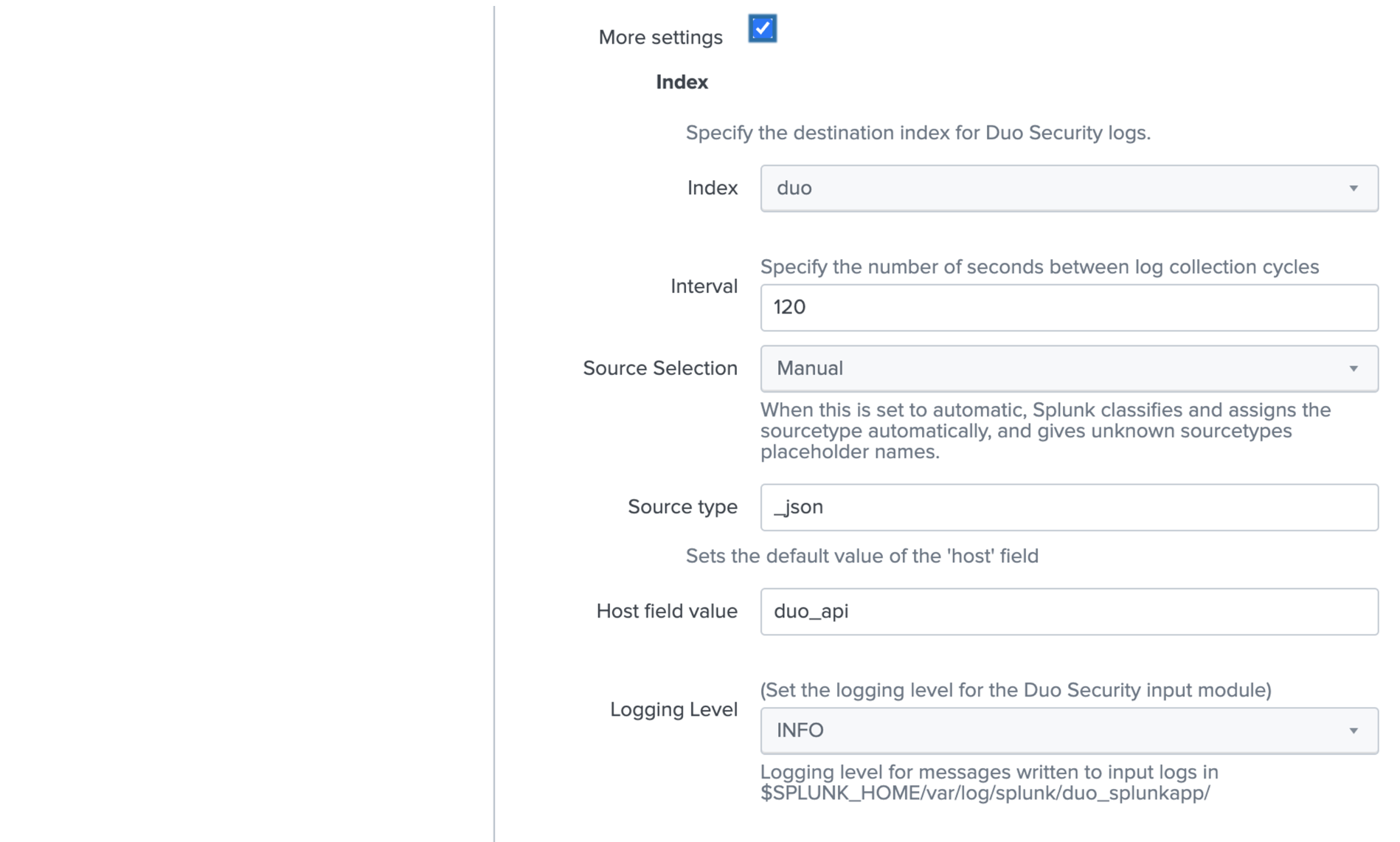In this detailed image, we start at the top left corner where the words "More Settings" are displayed. To the right of "More Settings" is a blue box containing a white checkmark. Directly below, there is a subsection titled "Index." Beneath the title, the text reads, "Specify the Destination Index for Duo Security Logs." Following this, the word "Index" appears again, alongside a large rectangular box on its right. Inside the box, the word "Duo" is positioned on the far left, while a down arrow is found on the far right.

Moving down, a similar layout is presented but this time with the title "Interval." To the right of "Interval" is another rectangular box holding the value "120." Below the "Interval" section, the title "Source Section" is displayed. Adjacent to this, within a box, the word "Manual" is printed. Underneath, an explanatory note clarifies, stating, "When this is set to Automatic, Splunk classifies and assigns the source type automatically and gives unknown source types placeholder names."

Continuing below, there is a sequence listing "Source Type," "JSON," "Host Field Value," and "Duo API." The final row is labeled "Login Level" with a box to the right stating "Info." Just above this row, there's an instruction mentioning, "Set the Login Level for the Duo Security Input Module," and below, a brief note: "Login Level for Messages."